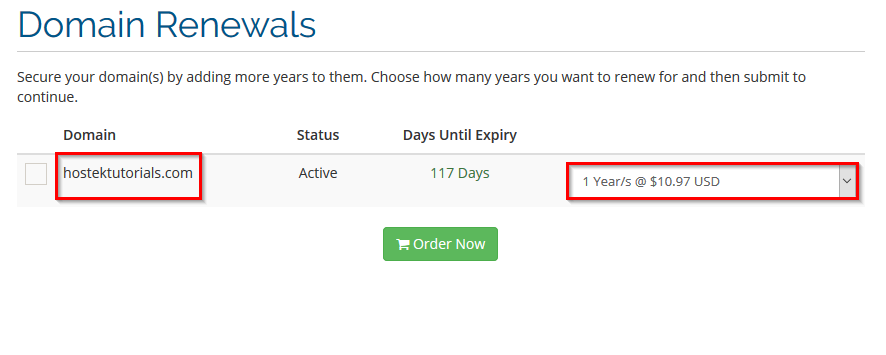This image captures a partial section of a website focusing on domain renewals. At the top of the section, the header "Domain Renewals" is prominently displayed, separated from the subsequent content by a line. Below this, a succinct instructional paragraph reads: "Secure your domain(s) by adding more years to them. Choose how many years you want to renew for and then submit to continue."

Following the paragraph, the content is organized into a structured table. The table has the headings "Domain," "Status," and "Days Until Expiry." The "Domain" heading is highlighted in bold black text. Directly beneath these headings, a series of organized elements are displayed:

- On the far left, an empty checkbox is available for selection.
- Adjacent to the checkbox, a red-outlined box contains the domain name "hostektutorials.com."
- To the right of the domain name, under the "Status" column, the word "Active" is shown.
- Further to the right, the "Days Until Expiry" column indicates "117 days."
- Adjacent to the days count, a long rectangular box with a red outline lists the renewal option as "1 year's at $10.97 USD" accompanied by a dropdown arrow for selecting different renewal periods if offered.

Beneath this table entry, a green "Order Now" button is prominently displayed, featuring a shopping cart icon, inviting users to proceed with the domain renewal purchase.